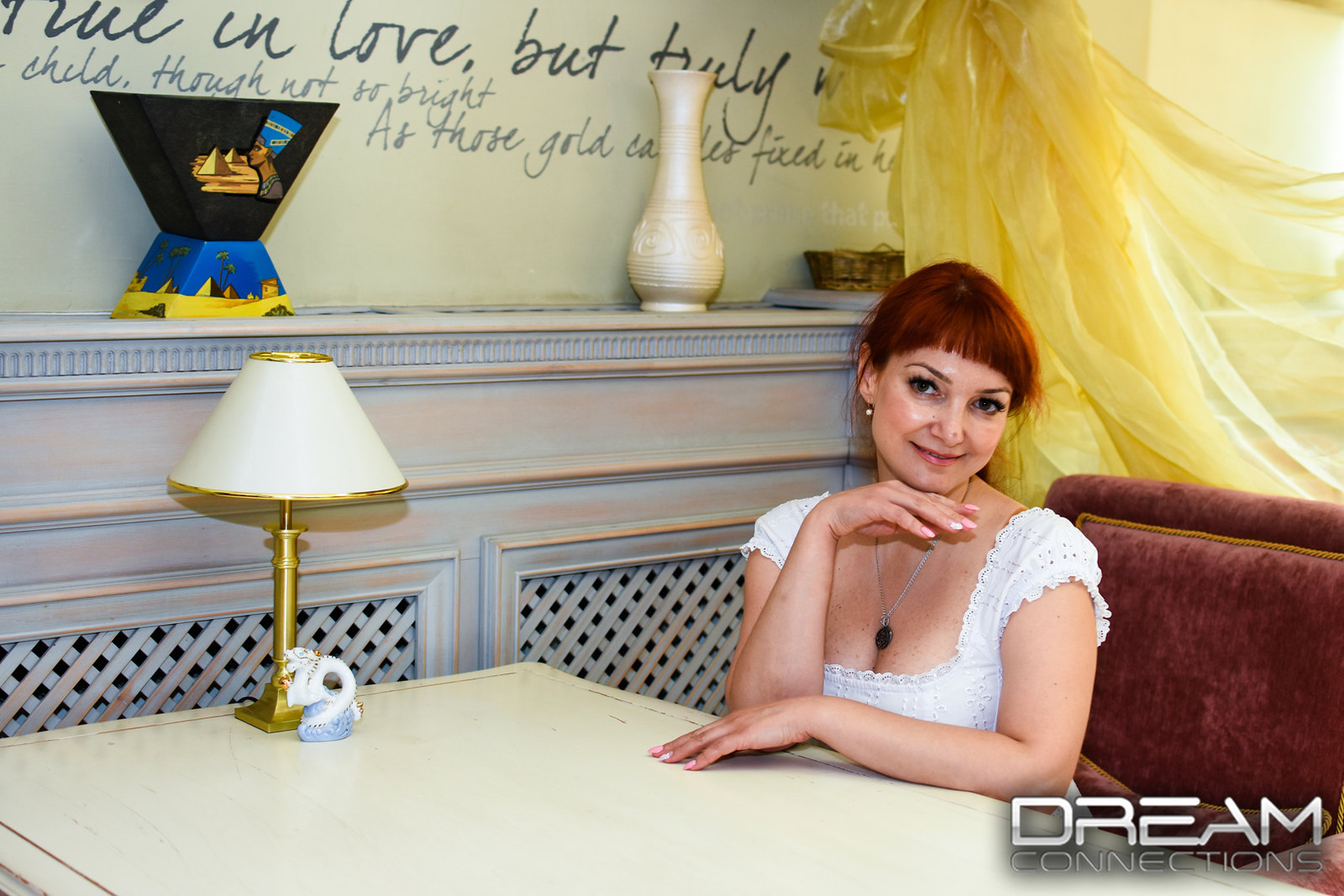This horizontally aligned rectangular photograph depicts a woman with reddish-brown hair, pulled back with bangs, smiling at the camera. She is seated in a booth or sofa at a white table, resting her chin on her hand while her other arm is laid on the table in front of her. The booth she sits in is either a brown or burgundy color, possibly with gold trim, or a red or purple shade. She is wearing a white blouse or dress and a necklace with a black pendant. Her nails appear to be painted white and pink.

To the left side of the table sits a small lamp with a gold base and a white lampshade, also trimmed with gold. Behind her, the white wall features a shelf with a vase and some writing, partially obscured by other items. The visible text reads "true love" and partially, "but truly child." Additional elements include a small figurine of an Eastern dragon, colored white and resting on a blue cloud, also on the table.

Above her, a yellow curtain is visible. In the lower right-hand corner of the image, large gray uppercase text states "DREAM CONNECTIONS." The image overall carries a sense of warmth and intimacy, likely associated with the Dream Connections website or service, emphasizing themes of love and connection.